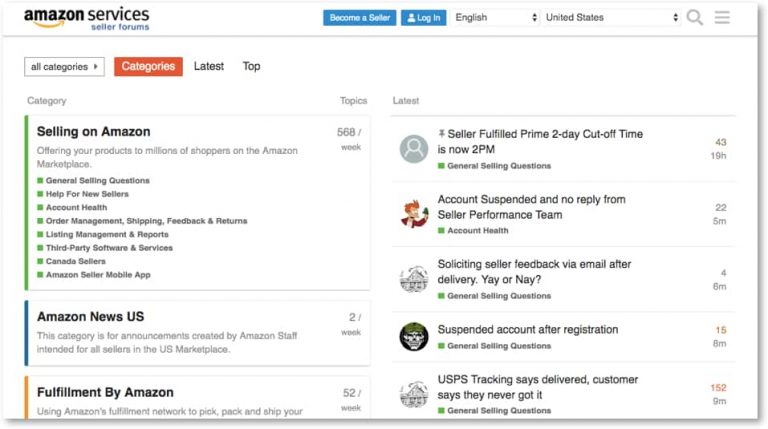**Detailed Caption:**

This image is a screenshot of the Amazon Services Seller's Forum interface. In the upper left corner, the page prominently displays the text "Amazon Services Seller's Forum" alongside the Amazon logo. Centered at the top, there are blue, clickable links labeled "Become a Seller" and "Log In." Adjacent to these, a language selection dropdown is preset to English, and the location is set to the United States. A magnifying glass icon indicates the presence of a search bar, while a three-line horizontal menu icon suggests more options are available.

Below these elements, there are various navigation categories labeled "All Categories," "Blue Categories," "Latest," and "Top," with the "Categories" tab highlighted in orange. On the left side of the interface, a section marked "Selling on Amazon" is displayed in bold text. Below this heading, several green boxes are arranged vertically, each representing different clickable options for users.

Further down on the left side, another section titled "Amazon News U.S." features a distinctive black bar on its left side. This section highlights "Fulfillment by Amazon" prominently in orange text. On the right side of the screenshot, a column titled "Latest" lists various forum topics, each accompanied by an icon. One highlighted topic is "Seller Fulfilled Prime 2-Day Cut-Off Time is now 2 p.m.," and each topic entry displays its posting time, the number of replies, and its category represented in a little green box.

This clear and organized interface facilitates easy navigation and accessibility for sellers seeking information, support, and community interactions on Amazon's platform.